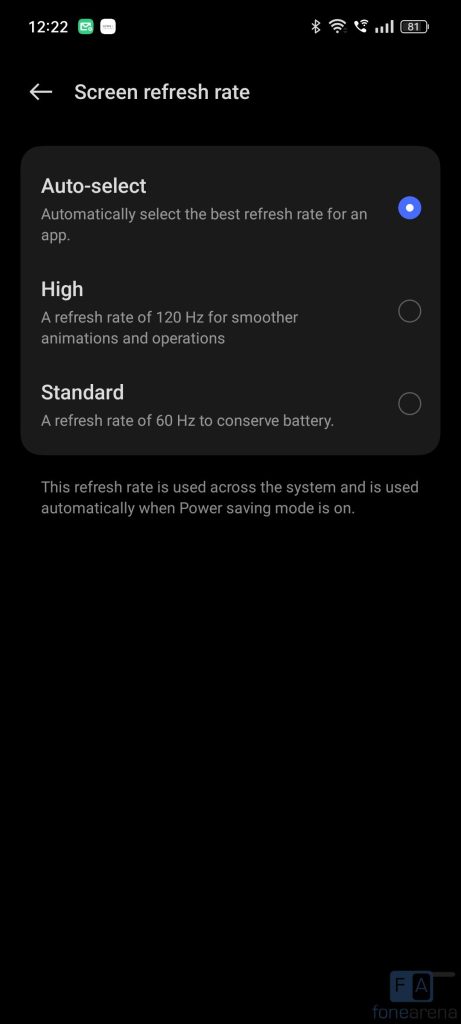In this image, we observe a user interface screen set against a black background. At the top of the image, the time is displayed as "12:22," accompanied by a green icon and a white icon to its right. A left-pointing arrow is visible, indicating a navigation option back to the previous screen, and the words "Screen Refresh Rate" are prominently displayed. 

Below this header section, there is a large box titled "Auto Select," which features an option to automatically select the best refresh rate for an application. Within this box, there is a smaller blue icon with white text centered within it.

Further down, the interface provides two distinct refresh rate options:
1. **High:** This option offers a refresh rate of 120 Hz for smoother animations and operations. This option has an associated empty circle, indicating it is not currently selected.
2. **Standard:** This option offers a refresh rate of 60 Hz, designed to conserve battery life. Similarly, it features an empty circle, signifying it is also not selected at the moment.

The screen informs the user that this refresh rate setting is applied across the system and will be automatically utilized when power saving mode is enabled. Below these details, the screen remains empty until the very bottom right corner.

In the bottom right corner, there is a white box containing the letter "F," next to a smaller black box with the letter "A." Beneath these icons, there is some unreadable text.

Overall, this interface allows users to choose between automatic, high, or standard refresh rate settings to optimize their device's screen performance and battery usage.